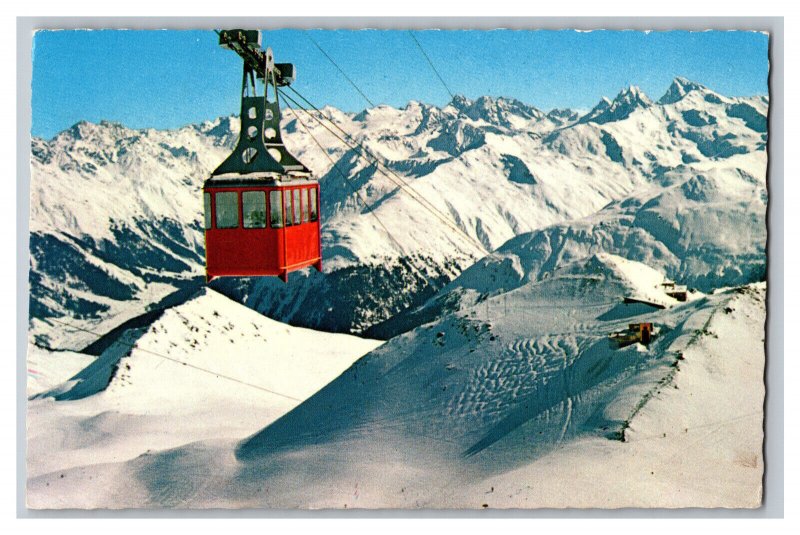This photograph, reminiscent of a postcard with its torn edges affixed to a gray card, depicts a red gondola ascending a snowy mountain. The gondola, a red box with clear windows and a black roof, is suspended from gray and black pulleys attached to a series of wires. The viewpoint is from above, looking down the mountain towards the gondola station below, surrounded by snow-covered terrain. At the base of the mountain, two houses can be seen – one red and the other appearing white, possibly covered in snow. Small figures, barely distinguishable, are seen walking in the snow, adding scale to the vast, wintry landscape. The entire scene is set against a backdrop of clear blue sky, enhancing the clarity and beauty of the snowy expanse.